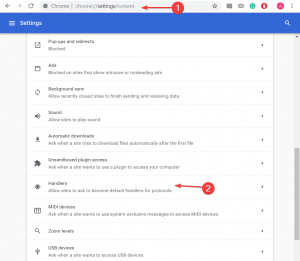A person is navigating through the settings menu on their laptop or computer using Google Chrome. The settings screen has a left-pointing arrow, indicating the ability to go back, but the right arrow is faded, implying that forwarding is not possible. To the right, there's a refresh button and a search bar.

The screen prominently displays the Google Chrome settings header. An arrow emerges from the right side, pointing left, and another arrow is accompanied by a circle with the number '1' inside. Further to the right, there is a star icon, potentially for bookmarking, and a folder or a common emoji.

A green icon with white lettering, possibly representing the Opera settings, can be seen. A username, abbreviated as "A," is displayed near the top. Underneath the search bar, which contains the word 'settings,' a blue horizontal bar spans across the screen. The interface includes a series of white horizontal lines to the right, resembling a menu icon, with a magnifying glass icon underneath.

Below these elements, various clickable options are listed, such as background synch settings, automatic downloads, and plug-in settings. Handlers are also mentioned, alongside another arrow pointing to the left with the number '2,' possibly indicating different subsections like devices, zoom levels, and USB devices. Each setting category has an arrow to the right, allowing users to delve deeper into specific options or features. The screen's pixelation poses some readability challenges, particularly when zoomed in.